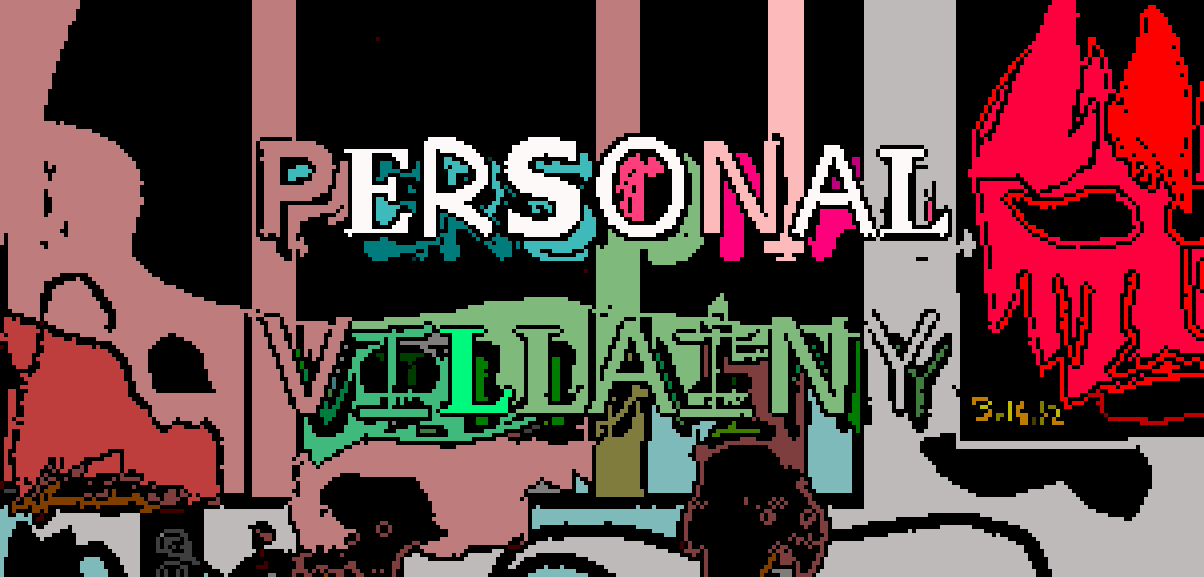The image features a vibrant and colorful digital artwork set against a predominantly black background. At the center of the image, the bold text "PERSONAL VILLAINY" is displayed in varying colors: the letters "P," "N," "V," and "Y" are slightly purple, while "E-R-S-O" are white, "A-L" are also white, and the remaining letters "I-L-L-A-I-N" are green. On the right side of the image, there is a striking red form outlined in black, resembling a mask or face with eye slots and horns, adding a dark, almost sinister element. The left side of the composition features three vertical pastel stripes, balancing the overall layout. The poster is further detailed with a date, reading "3-14-12," suggesting perhaps a specific event or creation date. This imaginative and slightly ominous artwork titled "Personal Villainy" combines dark themes with an explosion of colors including oranges, rosy pinks, and various shades of greens, conveying a complex mix of emotions and artistic expression.